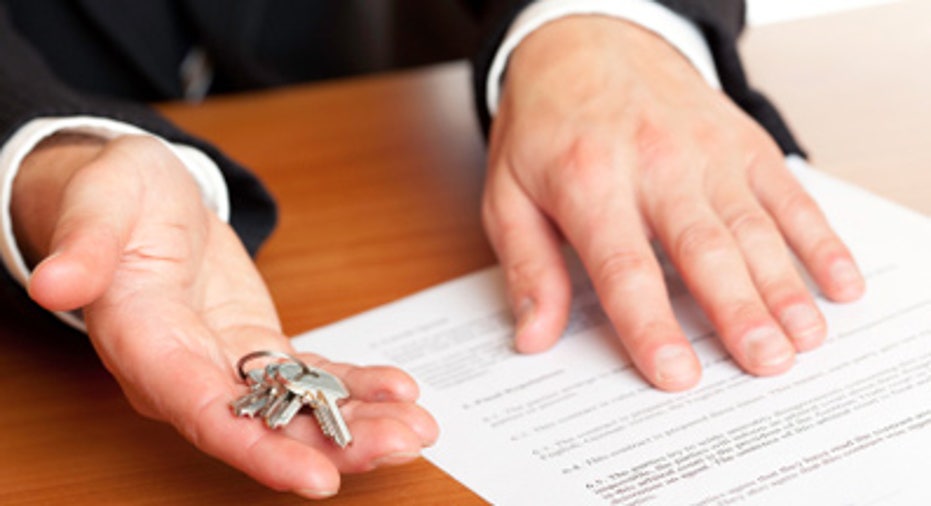The image captures a close-up view of a scene involving a Caucasian male engaged in what appears to be a business transaction. The man's hands are prominently displayed on a wooden table. He is wearing a black suit with white shirt sleeves peeking out. On the table, under his left hand, lies a sheet of paper that appears to be a contract or legal form. His right hand is outstretched towards us, holding a set of three silver keys, suggesting that the keys are being offered as part of the transaction. The composition of the photo emphasizes the imminent exchange, highlighting both the contractual document and the keys, indicating a formal and important handover, potentially related to real estate.